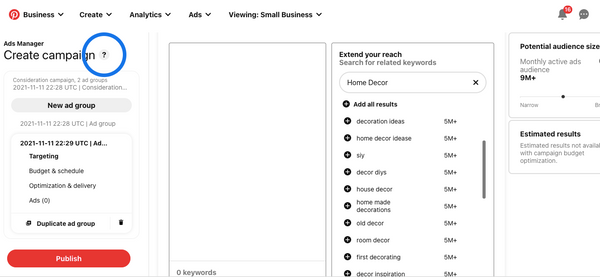The image displays a detailed interface of the Pinterest Ads Manager.

1. **Header:**
   - In the upper left corner, the Pinterest logo is prominently featured as a red circle with a white 'P'.
   - Following the logo, a black bold font menu with pull-down options lists "Business," "Create," "Analytics," "Ads," and "Viewing: Small Business."
   - To the right of these menus are some icons.

2. **Main Section:**
   - On the left side, there's a heading in black bold font that reads "Ads Manager".
   - Directly beneath this heading, in a larger font, it says "Create Campaign".
   - Below this, there's a bright blue circle with a white center, featuring text elements from "Create Campaign". The outer ring is bright blue with the characters "GN" and a question mark '?' visible within the ring.
   - Some gray text, which is too light to read, follows this element.
   - Continuing downwards, there's a gray horizontal oval with "New Ad Group" in black bold font.
   - Below this, various sections labeled with black regular font include "Dates," "Targeting," "Budget and Schedule," "Optimization and Delivery," and "Ads".
   - At the bottom of this section, in black bold font, it says "Duplicate Ad Group."
   - Adjacent to this, there's a rectangular, red, horizontal oval button labeled "Publish" in white font.

3. **Second Column (Central):**
   - This column is a vertical rectangular area outlined in light gray.
   - The body of this section is empty, with "Zero keywords" noted at the bottom left-hand side.

4. **Third Column (Right):**
   - At the top, in black bold font, it says "Extend Your Reach".
   - Beneath this, in gray, it reads "Search for related keywords".
   - There is a search box with "home decor" entered and an 'X' on the right side.
   - Below the search box, keywords are listed with a plus sign (+) on the left of each. The list is headed with "Add All Results" in bold font, while other entries are in regular font. Keywords include:
     - Decoration ideas
     - Home decor
     - [Unreadable text]
     - Sly decor
     - Do it yourself
     - House decor
     - Homemade decorations
     - Old decor
     - Room decor
     - First decorating
     - Decor inspiration
   - Each keyword is followed by "5M+".

5. **Fourth Column:**
   - This section is slightly elevated and starts higher than the others.
   - In bold black font, it reads "Potential Audience Size".
   - Below this, in gray, it says "Mostly Active Ads Audience".
   - Further down in bold black font, it shows "9M+".
   - Later in the column, it states "Estimated Results" in bold black font, with a note in gray indicating "Estimated results not available with campaign budget optimization."

This visually detailed description encapsulates the key elements and textual components featured in the image of the Pinterest Ads Manager interface.